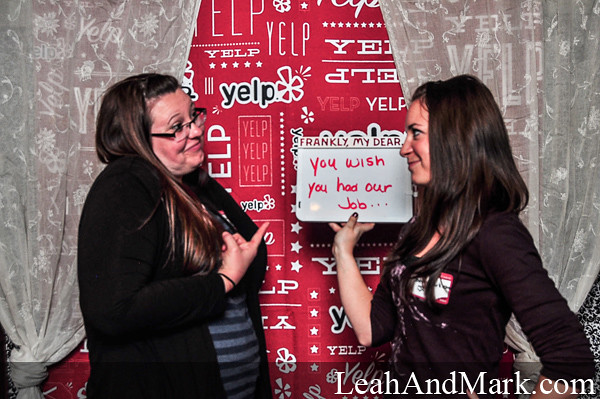This full-color indoor photograph, likely taken at an event, showcases two women engaged in a lively interaction. The woman on the left, slightly taller and wearing glasses, has long hair and is dressed in a black sweater layered over a blue and black striped shirt. She is pointing at a sign held by the woman opposite her while smiling and shrugging. This woman on the right, who has long black hair adorned with a distinct red name tag, sports a black top featuring decorative, scarf-like ropes. She is grinning broadly as she looks at her companion. The sign she holds reads, "Frankly, my dear, you wish you had our job..." capturing the playful tone between them. The backdrop consists of a red banner with "Yelp" repeatedly printed on it, framed by white, sheer curtains. At the bottom of the banner, the website "LeahAndMark.com" is visible.